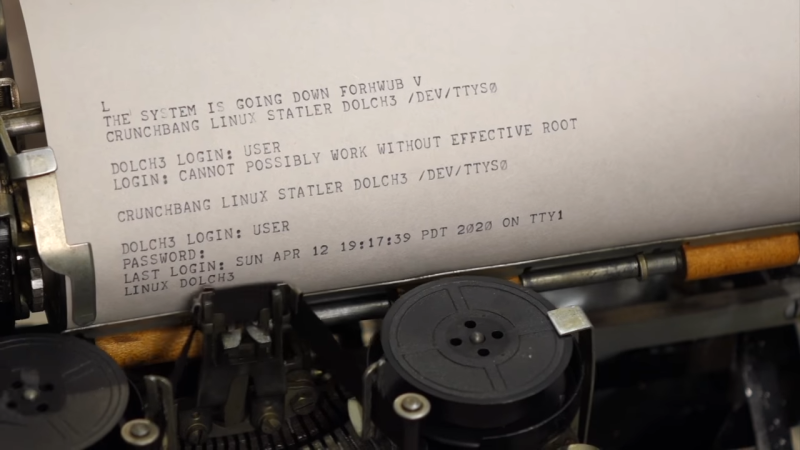The landscape-oriented image offers an evocative close-up of a vintage typewriter at work. The viewer’s attention is drawn primarily to the paper emerging from the typewriter, which is a slight off-white hue held taut by reflective steel clasps at the top and a brown or beige runner cylinder at the bottom. Prominently framed are two black spools with silver rivets.

The imagery is centered around the typed text on the paper, which is in an old-fashioned typewriter font. Upon close inspection, the first line contains a solitary "L." Below it, the text reads, "The system is going down 4 H W U B V." The subsequent lines reveal detailed computer system information, such as "CrunchBang Linux Statler Dolch 3" and "/dev/TTYSO." Additional lines include login prompts and system statuses, such as "Dolch 3 login: user," "login: cannot possibly work without effective root," "user password: nothing," and the last recorded login "Sunday, April 12th, 1917-39 PDT 2020 on TTY 1." The typeface also displays minor imperfections—some letters appear slightly faded, suggesting the typewriter ribbon did not imprint evenly.

Overall, this striking image combines elements of past and present technology, captured in a typewriter’s delicate keystrokes on a well-worn piece of paper.